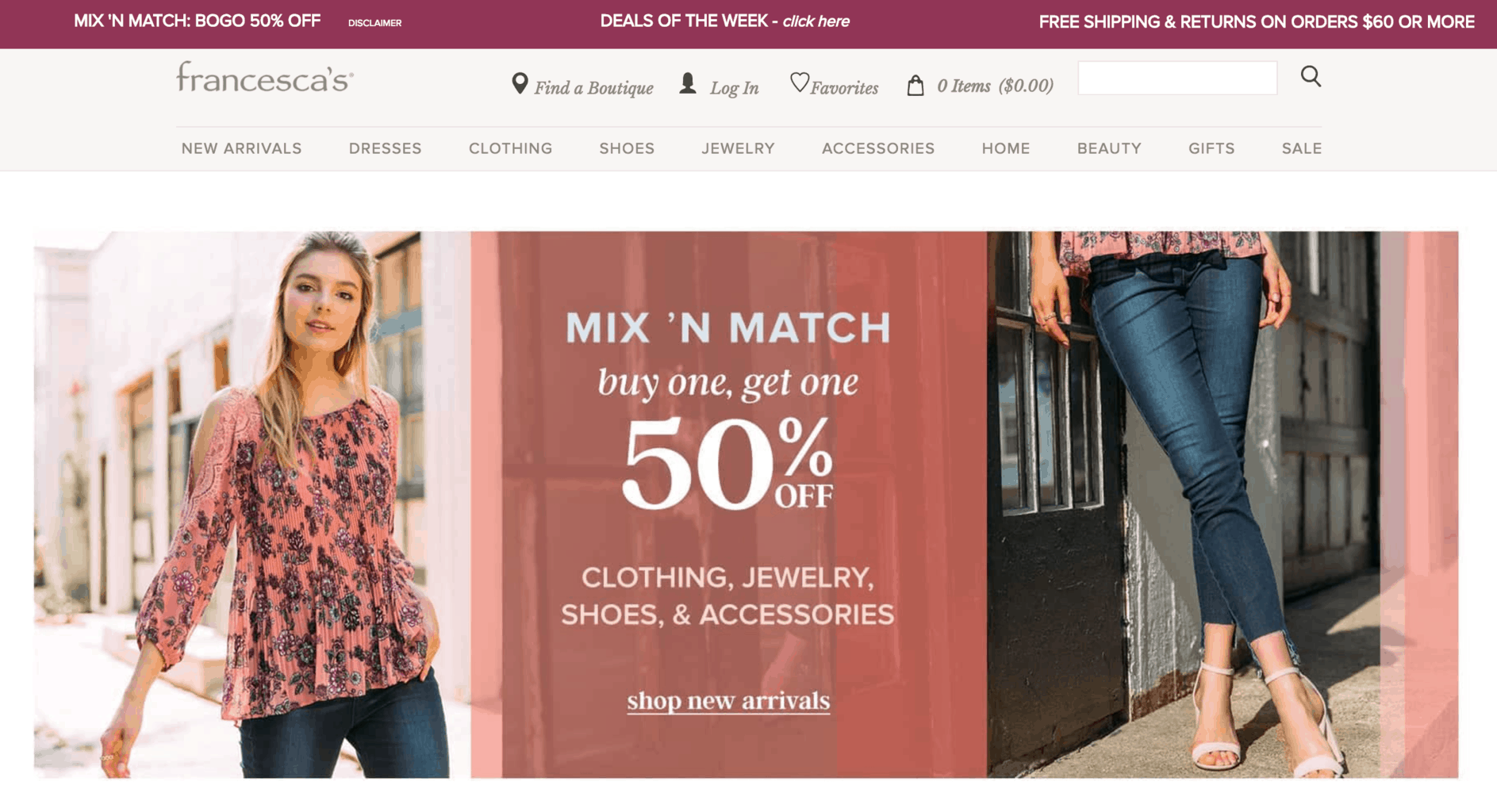The image showcases a promotional banner for Francesca's, a clothing and accessories retailer. At the top left, there is a prominent red bar with the text "Mix and Match, Buy One Get One 50% Off" featured. Additional text includes disclaimers like "Deals of the Week," "Click Here," "Free Shipping on orders $60 or more," and options such as "Find a Boutique," "Login," and "Favorites."

The primary focus of the image is a model positioned on the left side. She has long hair reaching her chest and is modeling a pink blouse adorned with black flowers, paired with tight-fitted blue jeans. She is styled with white shoes, including sandals and heels.

The background includes a rustic building, adding a textured backdrop to the scene. At the center of the image, text reiterates the offer: "Mix and Match, Buy One Get One 50% Off" on "Clothing, Jewelry, Shoes, Accessories." The text also encourages viewers to "Shop New Arrivals."

Overall, the image is well-lit, presenting clear visuals of the products. The model's pose against a wall on the right side adds a dynamic element to the composition, enhancing the appeal of the featured clothing items on Francesca's site.